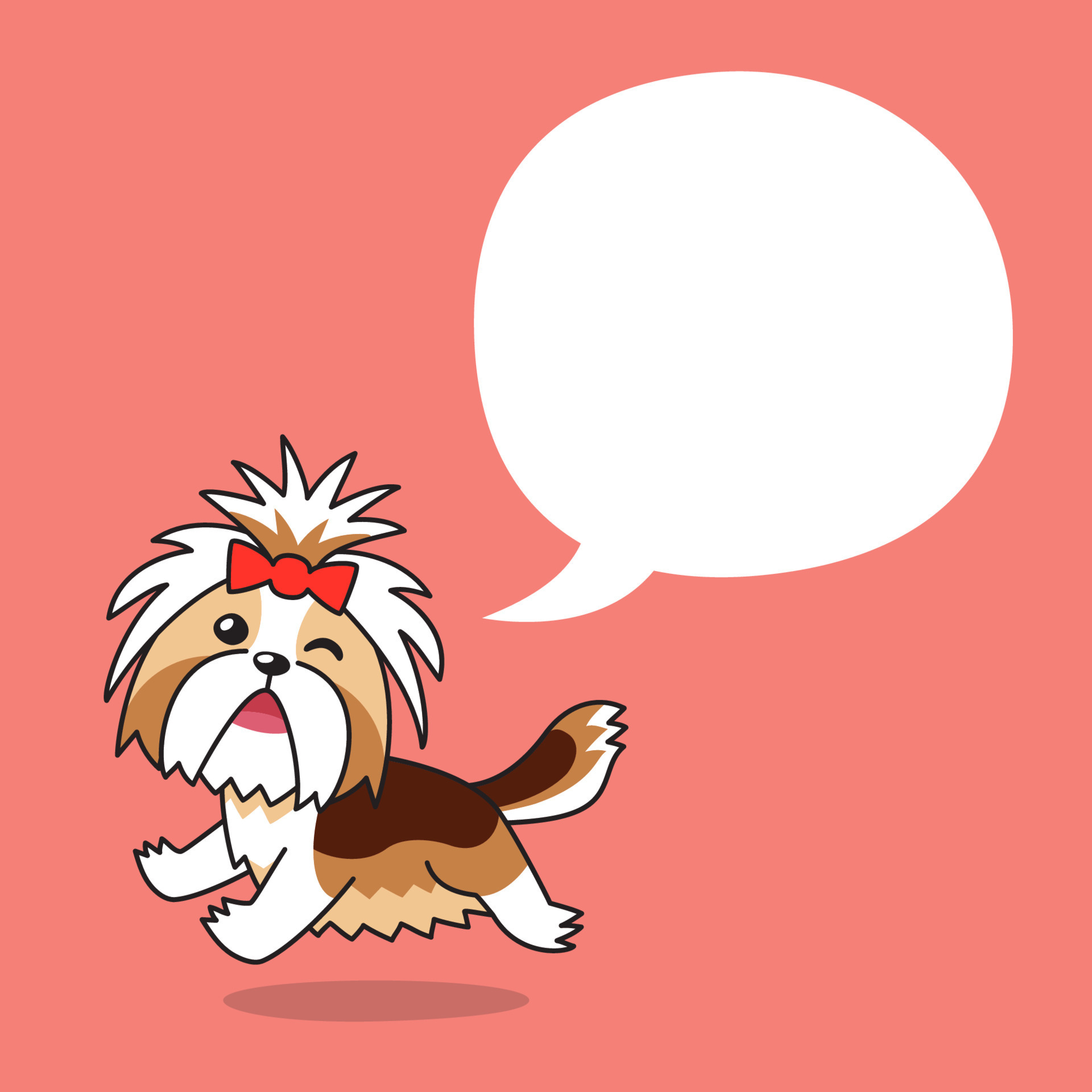The image depicts a computer-generated or digitally rendered scene with a small terrier dog as the central focus. The background is a pinkish-red or salmon color, and in the lower left corner, there is an expressive little terrier. The dog has a distinctive coat with shades of light brown, medium brown, and dark brown, along with little white legs and a white face. The dog's right eye is winking while the left eye is open, showcasing a playful expression. Additionally, there is a red bow perched on its head, adding a charming touch. The terrier is shown mid-stride, running to the left, with an oval shadow beneath suggesting motion through the air. In the upper right quadrant of the image is a large, white, empty quotation bubble, ready to be filled with text, making this a versatile piece for advertisement purposes.